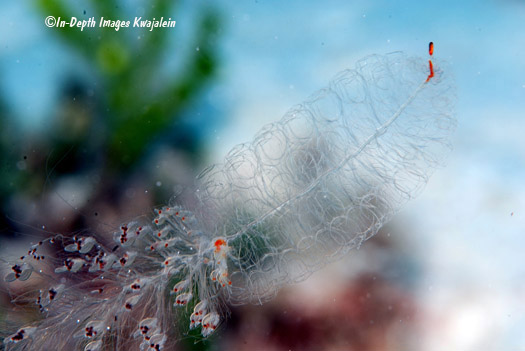This image, credited to In-Depth Images Kwajalein, depicts a beautifully intricate scene of nature in a delicate yet captivating manner. The background is subtly faded, hinting at what could be palm trees and other distant elements, creating a soft, blurred effect. The primary focus is on a large, almost transparent structure resembling a leaf or a flower. This natural form, although not made of plastic, showcases an ethereal material quality, highlighting its delicate and intricate design. This structure appears to be a seed dispersal mechanism, with one seed still clinging onto it while the rest have been released. The nearly translucent surface of this pod exhibits numerous empty spaces where seeds were once held, leaving behind tiny circular impressions. In the bottom left corner of the photograph, a few of these disbursed seeds are visible, resting gently. The overall composition of the image captures a moment of serene natural beauty and the intricate lifecycle of plant dispersal.